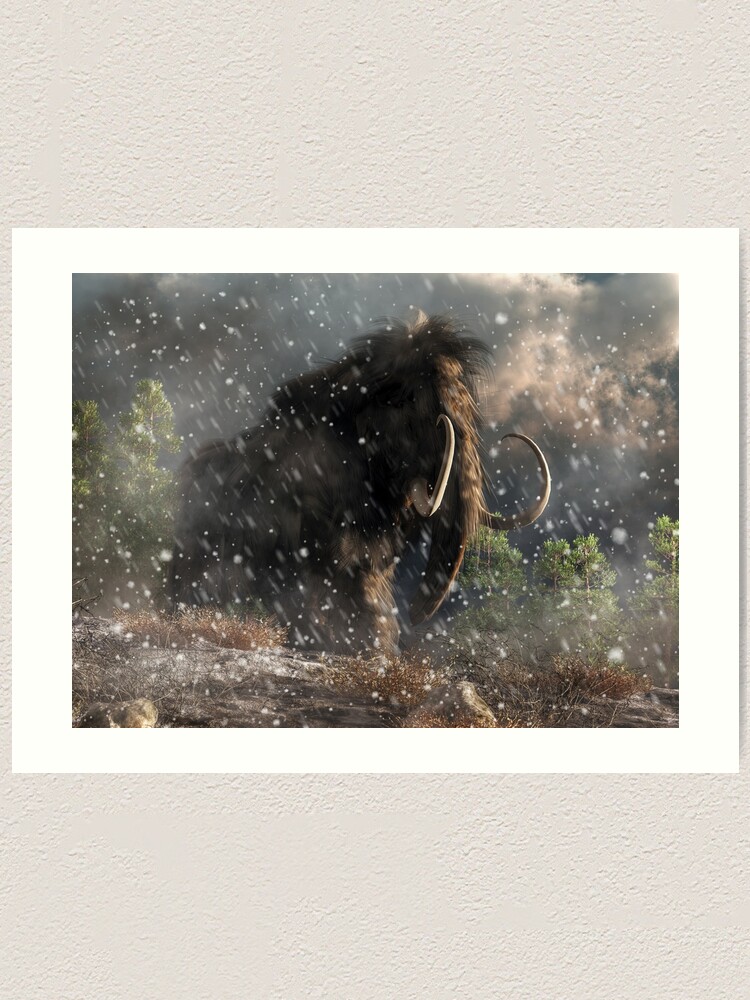The artwork displayed is a blurry, landscape-oriented painting of a colossal woolly mammoth with a dark brown, shaggy coat and prominent, curving white tusks. The mammoth is the central figure, towering over nearby green and tall pine trees. The background features a tempestuous gray sky filled with clouds, suggesting an ongoing snow or hail storm that envelops the entire scene. The ground below the mammoth shows traces of dirt amidst the storm. This striking image is encased within a simple white border and is hung against a very light tan wall, resembling a piece of paper rather than a traditional wooden frame.